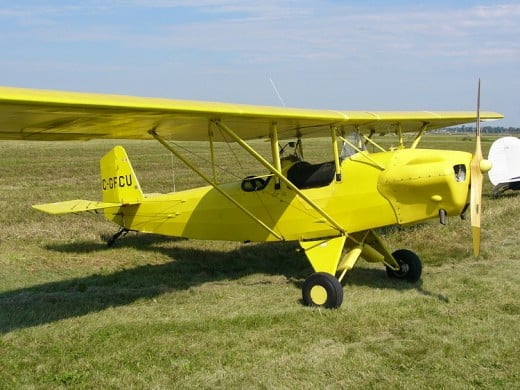The image showcases a small, old, yellow airplane situated in the center of a green grassy field, with a clear blue sky occupying the top third of the frame. The airplane, which features a unique design with an open cockpit and a small windshield, has a single wing running across its body. The bright yellow propeller is positioned at the front, while two black tires and yellow wheel wells are visible underneath the cockpit. Behind the airplane, there’s a white round object, and green trees can be seen in the distance. The plane’s tail displays the call letters C-GFCU. Casting a shadow on the grass, the yellow wings intersect the horizon where the sky and grass meet, adding a natural symmetry to the composition. Additional small stabilizer wings and a single wheel are located at the rear of the aircraft. The overall shape of the plane resembles a canoe with two girders extending from its body to either side of the wing.